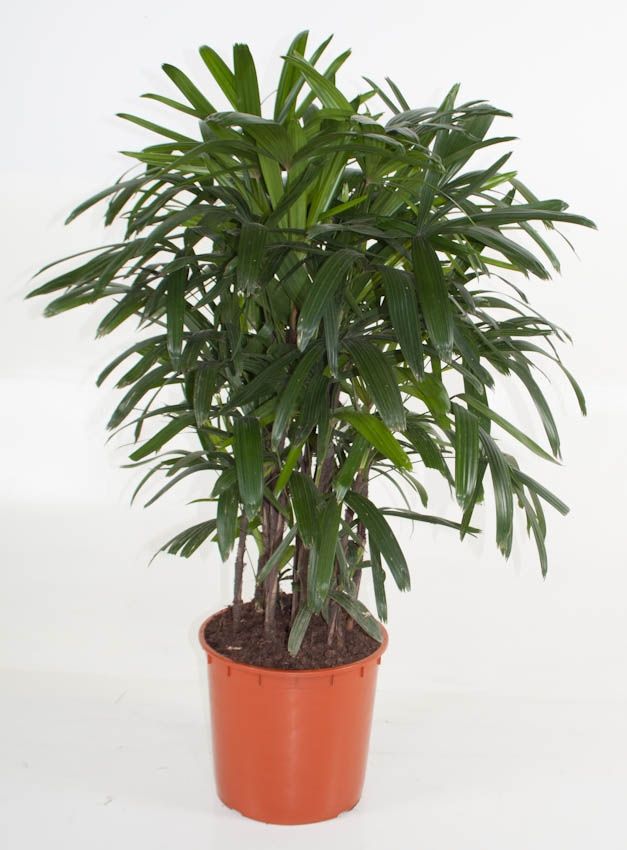This photograph showcases a tall, lush lady palm plant featured prominently in an indoor setting. The plant is contained within a medium-sized, light to dark burnt orange plastic pot filled with potting soil. Standing approximately three feet high, the lady palm displays a dense cluster of multiple stems adorned with long, draping leaves that resemble the shape and size of bananas. The rich, deep green foliage is a striking contrast against the off-white background, making it a perfect decorative element for indoor spaces such as an office. The setting is minimalist, with no identifying information such as dates or names, and the image dimensions are approximately three by five inches.